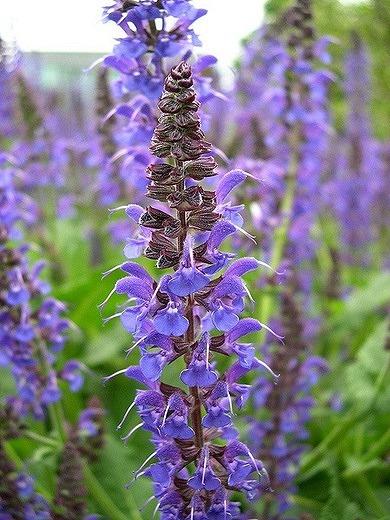This professional photograph captures a stunning close-up of a vibrant bluish-purple flower with bell-shaped petals, prominently in focus against a beautifully blurred background. The main flower stands tall on a long stalk, exhibiting rich hues that seem to change between blue and purple depending on the light. Some of the petals at the top appear shriveled or blackened, adding a touch of natural imperfection. Stretching out behind it is a vast field filled with more of these striking flowers, creating a sea of blue that extends to the horizon. Interspersed among the flowers are green grasses, stems, and leaves, contributing to the lush feel of the scene. The background also features blurred green trees, possibly coniferous, under a misty white sky, and in the far distance, a wooded hill can be faintly discerned. This pure nature shot, devoid of any text, beautifully showcases the flowers in their natural habitat.